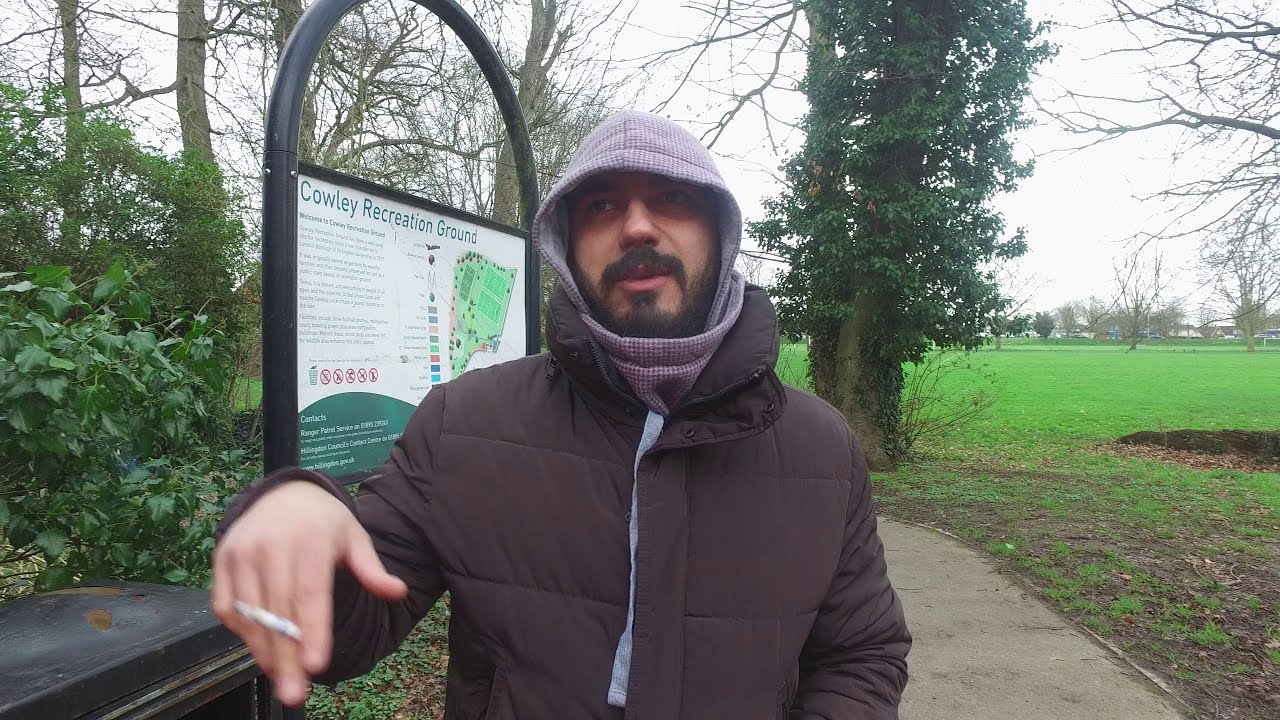A bearded man stands at the center of the image, leaning against a metal guard rail in a park area as he faces the camera. Clad in a buttoned-up brown quilted winter coat with a hood from his sweatshirt pulled over his head, he also has a cigarette nestled between his fingers in his right hand. His attire suggests a cold day. To his right stands a sign reading "Cali Recreation Ground," displaying a map detailing the park's amenities, such as tennis courts. The background reveals a vast expanse of green grass with trees, some barren and others with leaves, while a sidewalk begins at the bottom of the image and extends into the park. To his left, more trees and bushes are evident, completing the serene, verdant setting.